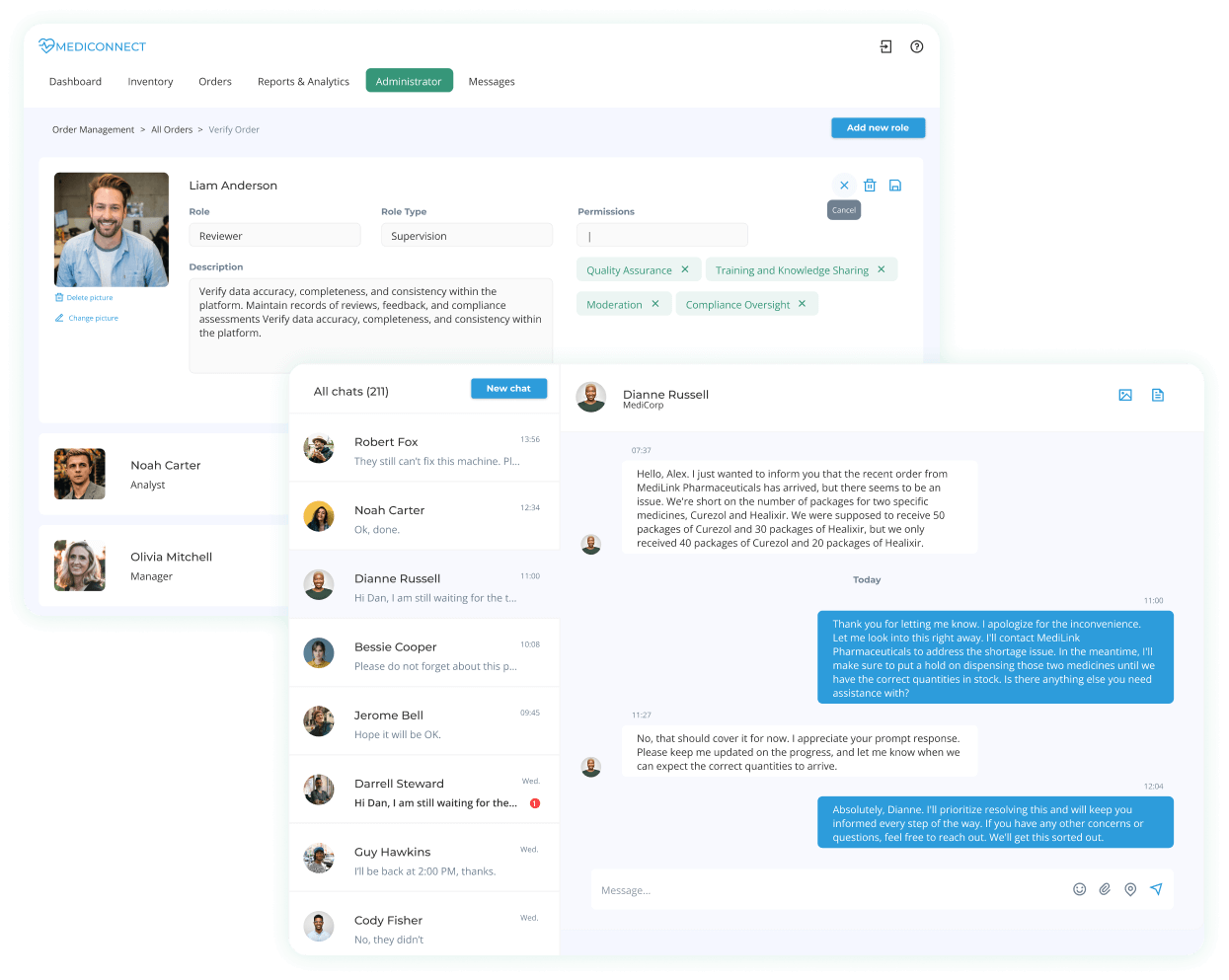**Detailed Caption:**

This image is a screenshot of a webpage from a platform called "MetaConnect," as indicated in the top left corner. Below the title, a navigation menu features several tabs including "Dashboard," "Inventory," "Orders," "Reports," and "Analytics." The "Administrator" tab is highlighted, revealing a sub-section labeled "Messages."

Beneath the navigation, the title "Order Management" is displayed, followed by options such as "All Orders" and "Verify Order." The main focus of the page is a profile photo of a smiling man named Liam Anderson, identified as a Role Reviewer with supervisory duties. His role description includes verifying data accuracy, completeness, and consistency within the platform, in addition to maintaining records of reviews, feedback, and compliance assessments. His name and role details are prominently displayed next to his photo.

To the left of this central content are two additional profile icons. One features a man named Noah Carter, an Analyst, and the other showcases a woman named Olivia Mitchell, a Manager.

Also displayed is a chat record listing "All Chats 211" with names such as Robert Fox commenting on ongoing machine issues, Noah Carter confirming a task completion, and Diane Russell questioning Dan about pending matters. To the right, Diane Russell's profile icon and name appear alongside a detailed text message. She informs a recipient named Alex about a delivery issue with an order from MediLink Pharmaceuticals. Specifically, the shipment was short by 10 packages of Curazol (40 instead of 50) and by 10 packages of Helixir (20 instead of 30). The message concludes with a response from the recipient promising to look into the issue.